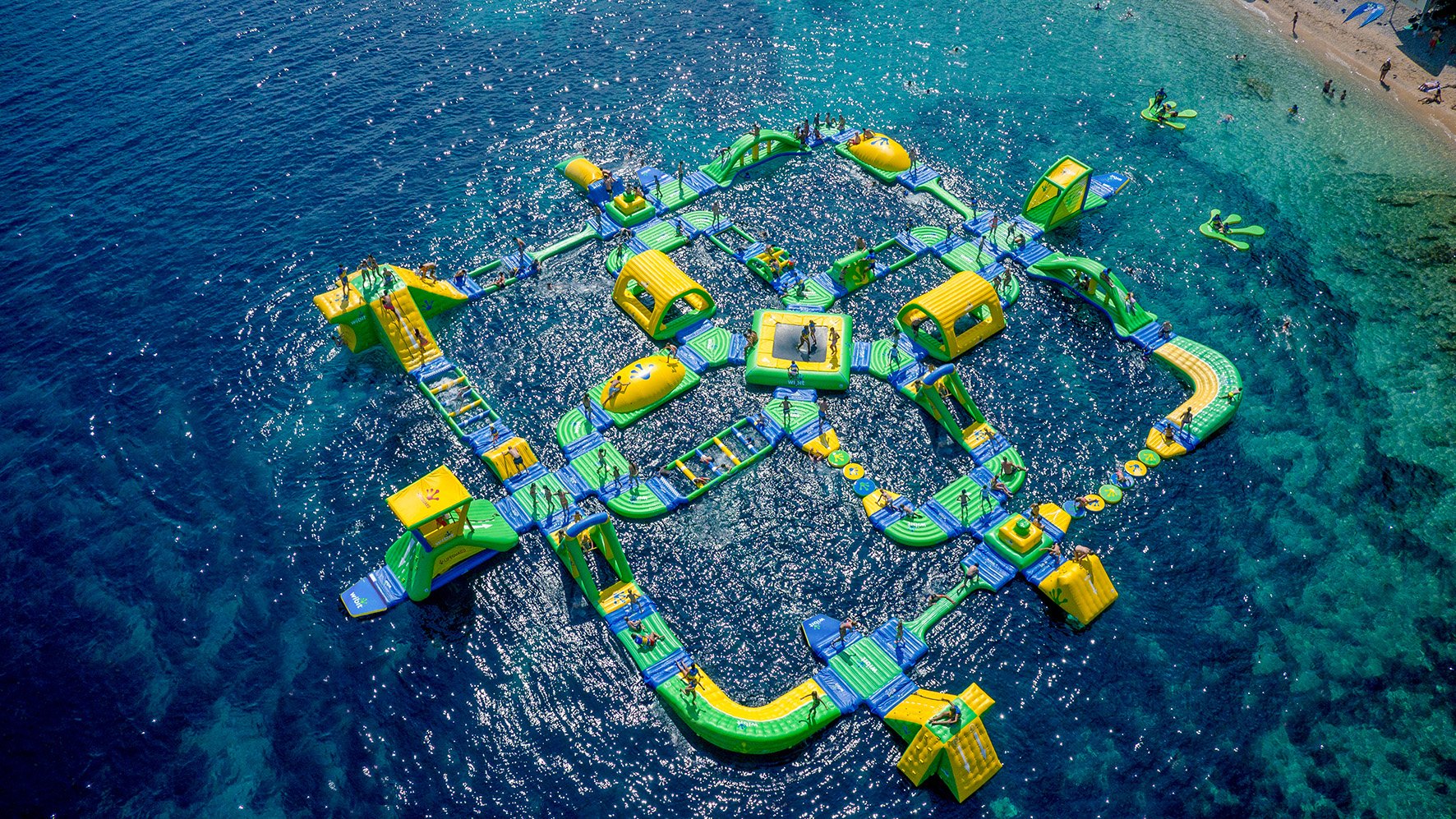Captured from the sky, this top-down image showcases a vibrant, expansive water playground situated just offshore in a stunning ocean environment. The playground is a large, interconnected network of inflatable structures, primarily colored in yellow, green, and blue. Centrally arranged in a square layout with a plus sign at its core, this floating playground features an array of shapes and activities. There are platforms, domes, slides, and trampoline-like areas. Additionally, some sections resemble air cushions for jumping, and others look like ball pits or steps. The playground floats atop the water, with the turquoise and dark blue hues of the ocean creating a beautiful backdrop.

In the top right corner of the image, a sandy beach is visible with people standing and walking along the shoreline. On the water playground itself, about 30 individuals, including children, are seen enjoying various activities, running, sliding, and being catapulted into the water from air mattresses designed to launch them skyward. The entire structure appears large, potentially around 100 feet by 100 feet, making it a massive floating attraction. The colors and arrangement of the inflatable pieces add a lively, inviting appearance to the scene, making it a dreamlike destination for endless fun in the sun.